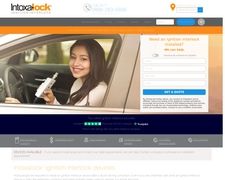The image depicts a website interface believed to be for a platform called "Interlock". In the upper left-hand corner, somewhat blurred but discernible, are the words "Into" followed by "Lock", the latter in orange font. Adjacent to these words on the right, there is an icon resembling a GPS marker. Below, a bar that appears to be a search function is visible, featuring a blue square icon.

The central section of the website showcases a media image featuring a woman who is smiling and facing the camera. She is holding an item in her hand, possibly a drink or a device, though it is not entirely clear.

To the right of the image, a highlighted orange font in the center of a box suggests an area designed for inputting various types of information. Below this section, four empty boxes are aligned side by side, likely intended for user input.

At the bottom of the interface, a blue-highlighted box is visible with some fine print text directly beneath it. This text is presumably additional information or instructions regarding the website’s usage or content.